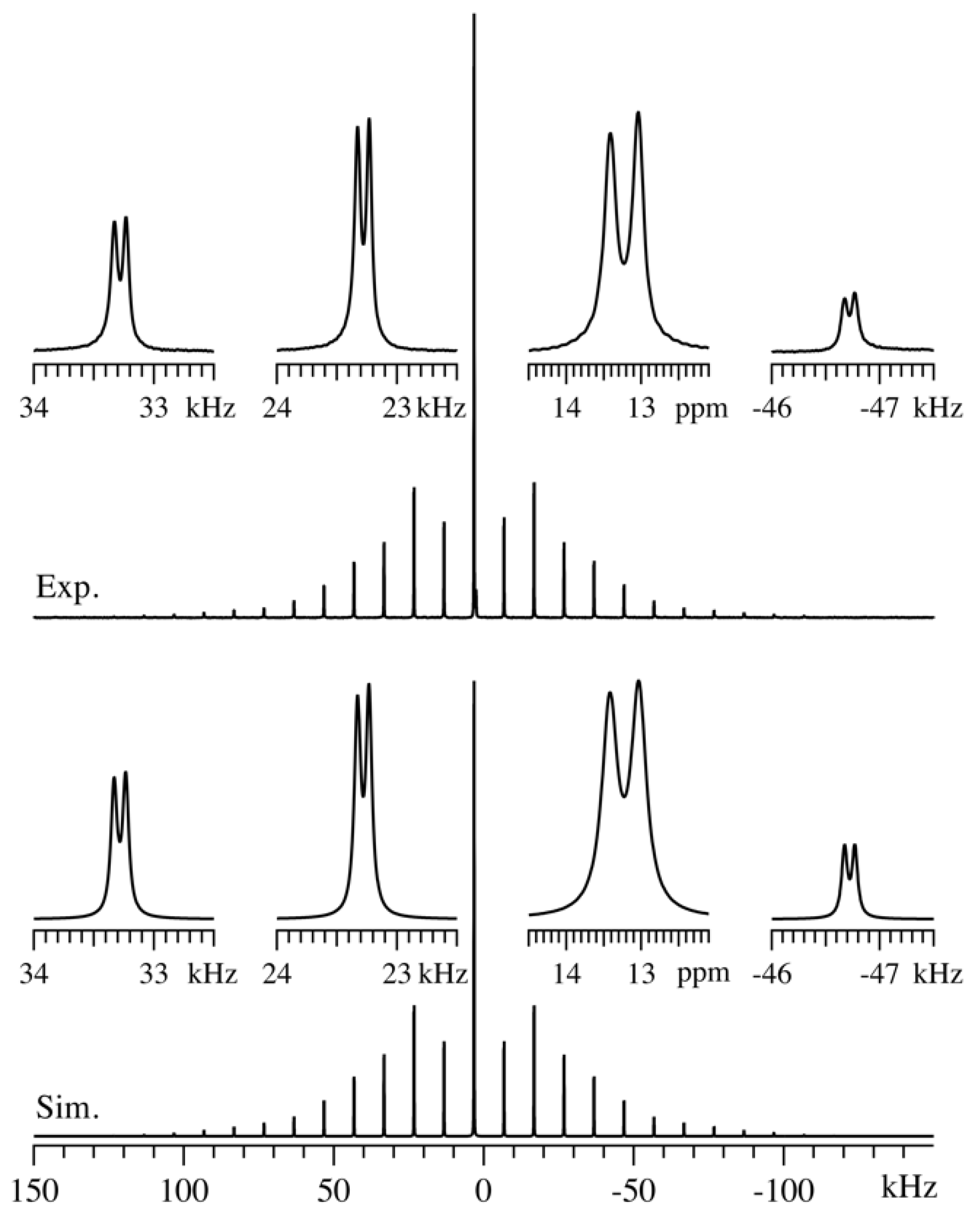The image displays a series of eight detailed graphs arranged in two rows, each meticulously rendered in black on a white background, resembling sound waveforms. The top row is labeled "EXP," and the bottom row is labeled "SIM." Each of the four graphs in the top row and their corresponding counterparts in the bottom row depict data measured in kilohertz (kHz) and parts per million (ppm). The first graph shows a parabolic pattern with a peak, measuring from 34 to 33 kHz. The second graph follows a similar pattern with values from 24 to 23 kHz. The third graph uniquely measures from 14 to 13 ppm, unlike the others. The fourth graph dips below the axis, ranging from -46 to -47 kHz. The bottom set's graphs mirror those above but are labeled "SIM," denoting simulated data. These graphs highlight specific increments marked along the horizontal axes, emphasizing variations at each point.